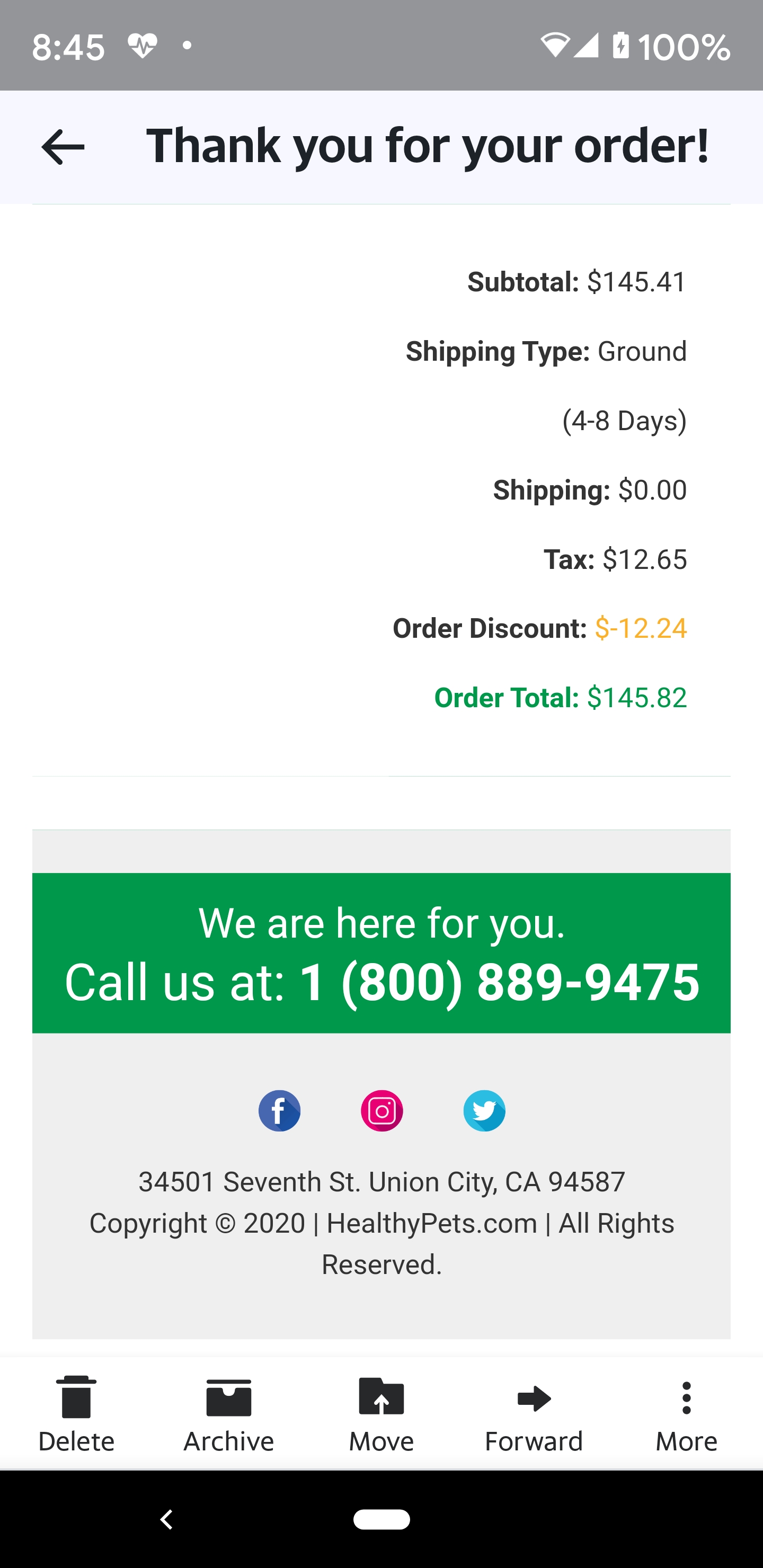A detailed screenshot captured from a smartphone displays a purchase confirmation for an order placed online. The confirmation message reads, "Thank you for your order," followed by an itemized list of charges including a subtotal of $145.41, shipping method via ground (4-8 days) costing $0, tax amounting to $12.65, an order discount of $12.24, and a final order total of $145.82.

At the bottom of the confirmation message, there is a green box with customer support information that says, "We are here for you, call us at 1-800-899-4755." Below this section, social media icons for Facebook, Instagram, and Twitter are displayed, along with the company's address: "34501 7th Street Union, California 94587." The footer also includes copyright information stating, "Copyright 2020, healthypets.com, all rights reserved."

The smartphone interface includes a menu bar at the bottom of the screen with options to delete, archive, move forward, or access more features. The status bar at the top of the screen shows the time, Wi-Fi signal strength, and battery life. Additionally, the phone features a home button at the bottom, accompanied by a black bar and a back button.

This comprehensive screenshot provides a clear view of the online order confirmation process on a mobile device, highlighting both the transaction details and the user interface elements.